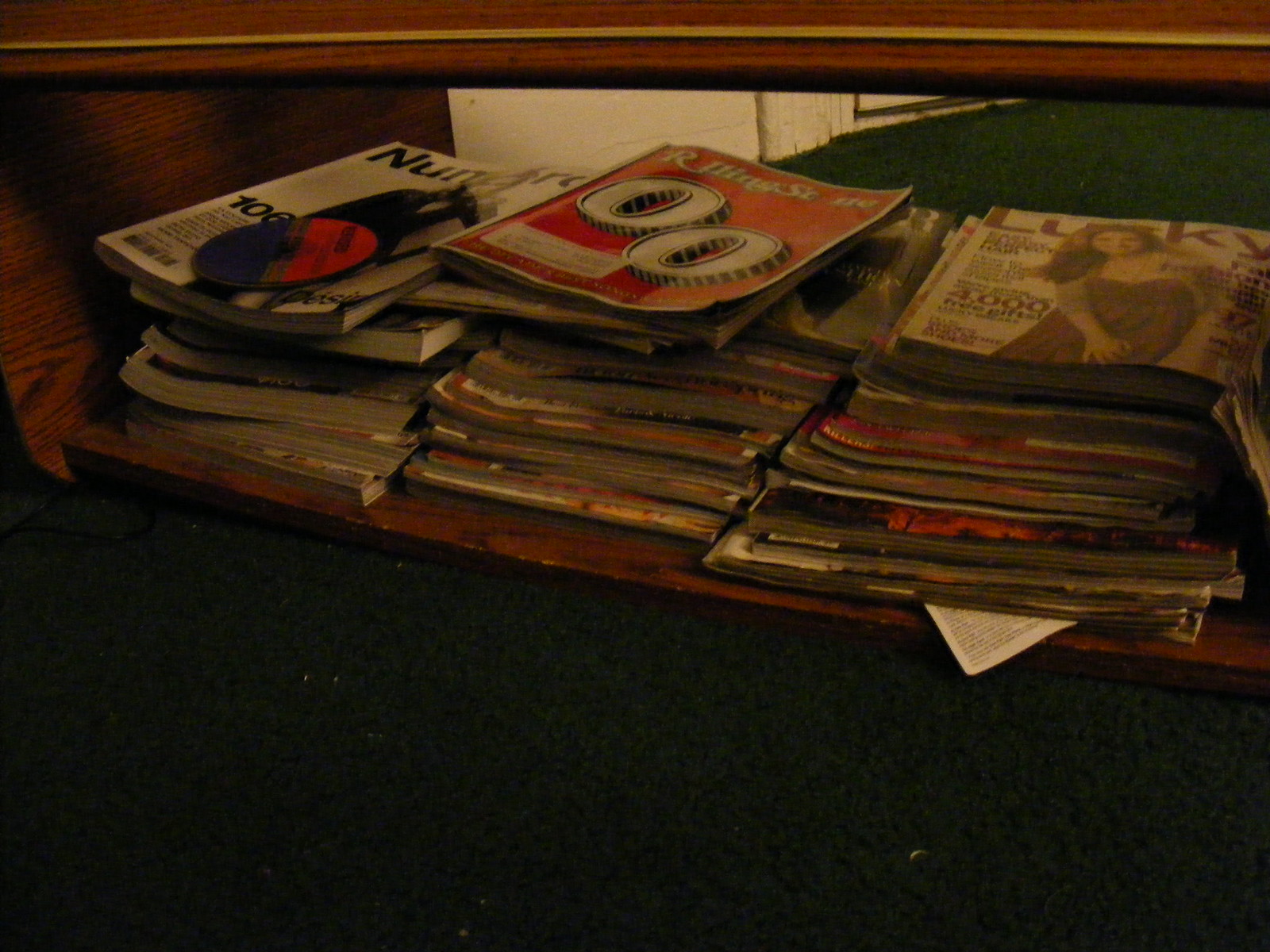In this dimly lit photo, a wooden shelf extending diagonally from the far right to the left side of the frame holds three disheveled stacks of magazines, each containing eight to ten or more issues. The leftmost stack features thicker magazines, possibly including catalogs. The center stack is topped by a red-covered issue of Rolling Stone, marked by white lettering and two large white zeros, with a visible subscription label at the bottom. On the rightmost stack, the top magazine is an issue of Lucky, featuring a Caucasian woman with long auburn hair in a red dress with a gray sleeve. The room around the shelf has a very dark green carpet and a white baseboard, adding to the overall dark ambiance of the scene.